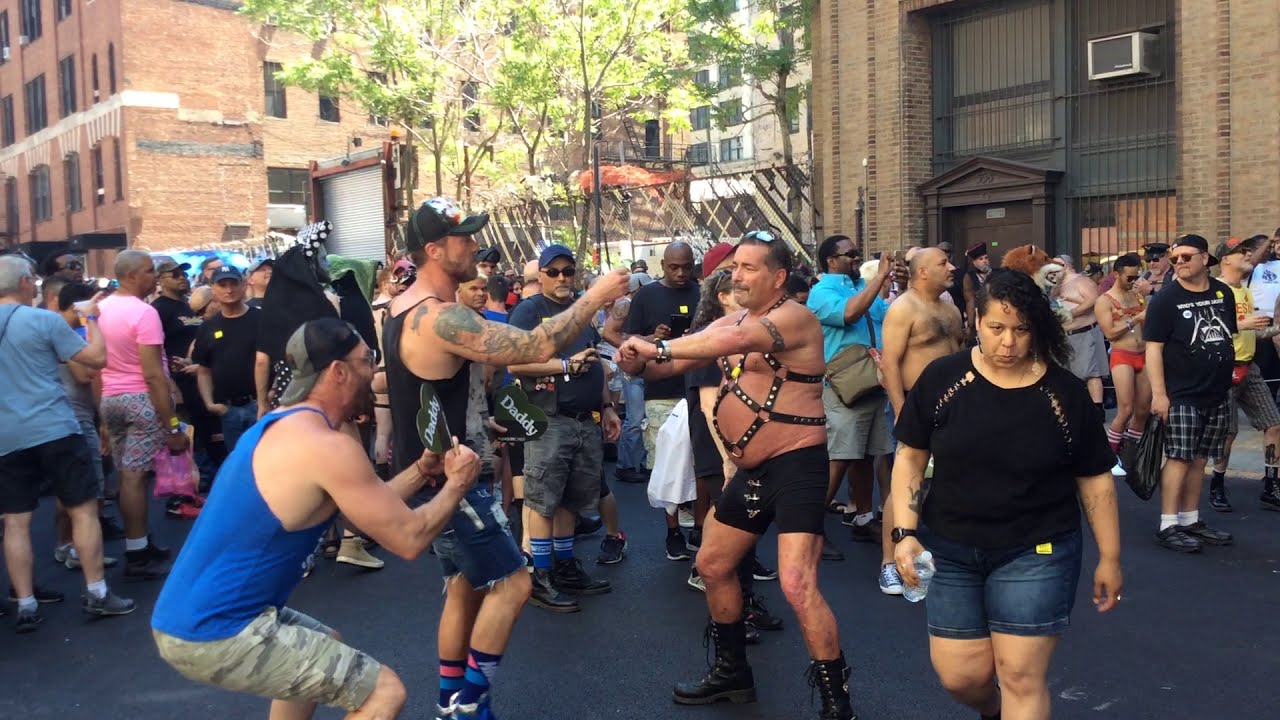In this vibrant, full-color photograph taken on a sunny day in a city, a lively scene unfolds at what appears to be a gay pride parade. The image, set against a backdrop of brownish brick buildings that rise up several stories high and are partially obscured by the dense crowd, captures the bustling activity of the event. Predominantly male participants of various ages are gathered outdoors, many of whom are engaged in different activities, suggesting a celebration of diversity and solidarity. 

At the center of the photograph, a shirtless Caucasian man draws attention, boldly adorned in an intricate black leather harness with studded straps, black leather shorts, knee-high black boots, and black lace-up sneakers. He wears sunglasses on top of his head and studded wristbands. This man energetically dances with another man, who sports a black tank top, a ball cap, heavily tattooed arms, jean shorts, and running shoes. 

Adding to the eclectic mix, a man in red panties and a bra appears on the right side of the image, while another individual in the lower left corner, dressed in a blue sleeveless tank top and camouflage shorts, crouches down, seemingly captivated by the dancers. He is holding green heart-shaped signs that read “Daddy.”

In the background, a woman with black hair, wearing a black short-sleeved blouse and blue jeans and carrying a water bottle, strides toward the camera with a serious expression. The scene is enriched by the presence of trees and the bustling foot traffic of the parade-goers. The lively and diverse atmosphere, punctuated by the unique and expressive attire of the participants, epitomizes the spirit and celebration of the gay pride parade.